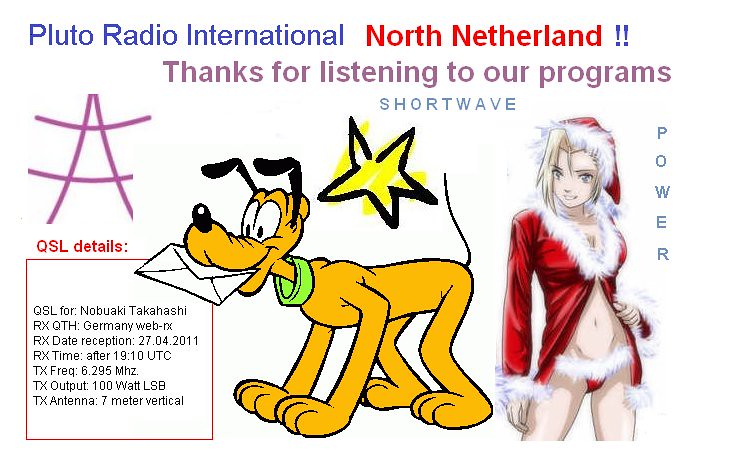The image features a white background with several elements, including text and cartoon drawings. Across the top, "Pluto Radio International" is written in blue, followed by "North Netherlands" in red, and beneath that, "Thanks for Listening to Our Programs" in purple, with "Shortwave" in blue. In the middle of the image is an illustration of Pluto the cartoon dog, colored yellow with black outlines and wearing a green collar, holding a letter in his mouth. Above Pluto is a scratchy drawn star with a black outline and a yellow scribbled center. To the right of Pluto is an anime character with blonde hair and light-colored eyes, depicted in a provocatively styled Santa outfit—a red jacket with white fluffy cuffs and bodice, only buttoned at the breasts, exposing her belly and thong-style panties which are also red with white fluff. The word "Power" is written vertically along the right side of this anime character. On the left side of the image is a purple symbol resembling the letter "A" with an extra horizontal line. Below this symbol, in red, is the text "QSL Details" followed by information in a red box, detailing QSL information including the name Nobuaki Takahashi, reception details from Germany, the date 27.04.2011 after 1910 UTC, transmission frequency 6.295 MHz, output power 100W, and a 7-meter vertical antenna.